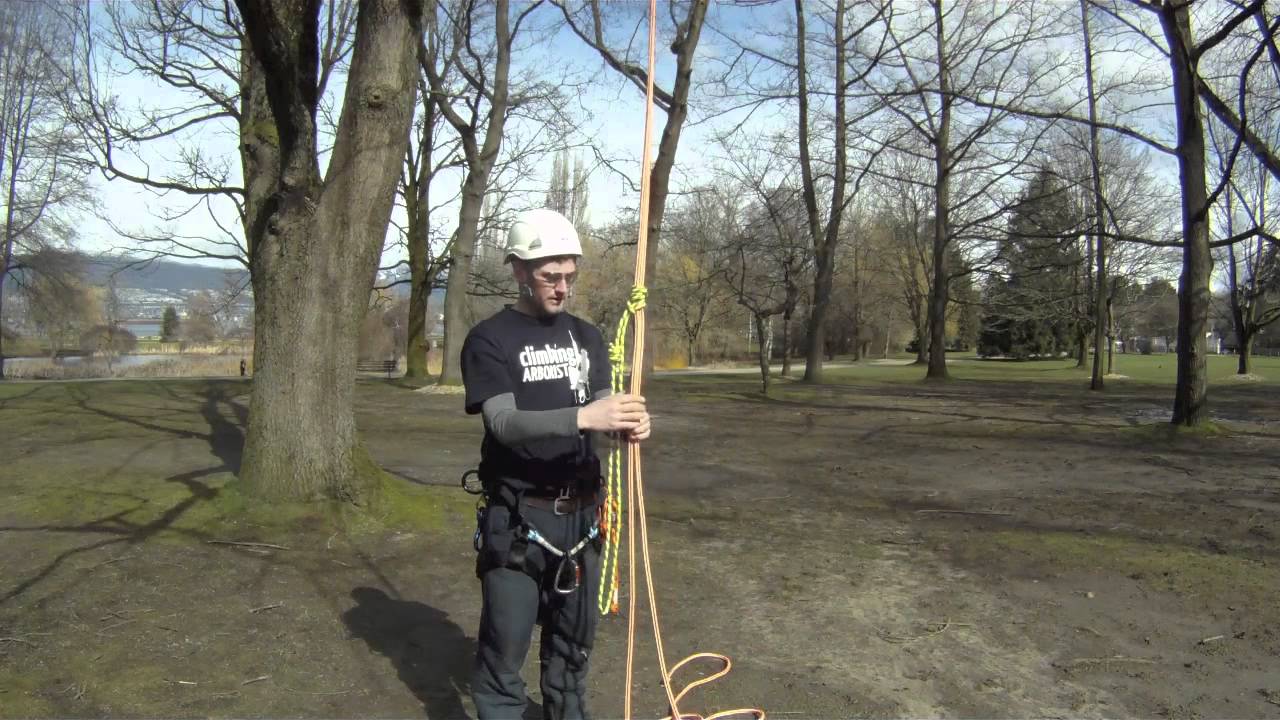A man, standing centrally in the image, is geared up for climbing in a sparsely wooded area, presumably a park during autumn or winter, as the leafless and somewhat scraggly trees suggest the off-season. He is dressed in a black t-shirt with "Climbing Arborist" printed in white over a grey thermal, black pants, and a white safety helmet. The ground appears mostly dirt, possibly due to recent heavy rain, with sparse grass and a visible walkway in the background. He is equipped with climbing gear, including yellow and orange ropes fastened to a harness around his waist, and seems to be preparing to ascend a tree branch just out of the frame. Behind him, a cityscape and a body of water stretch across the horizon.